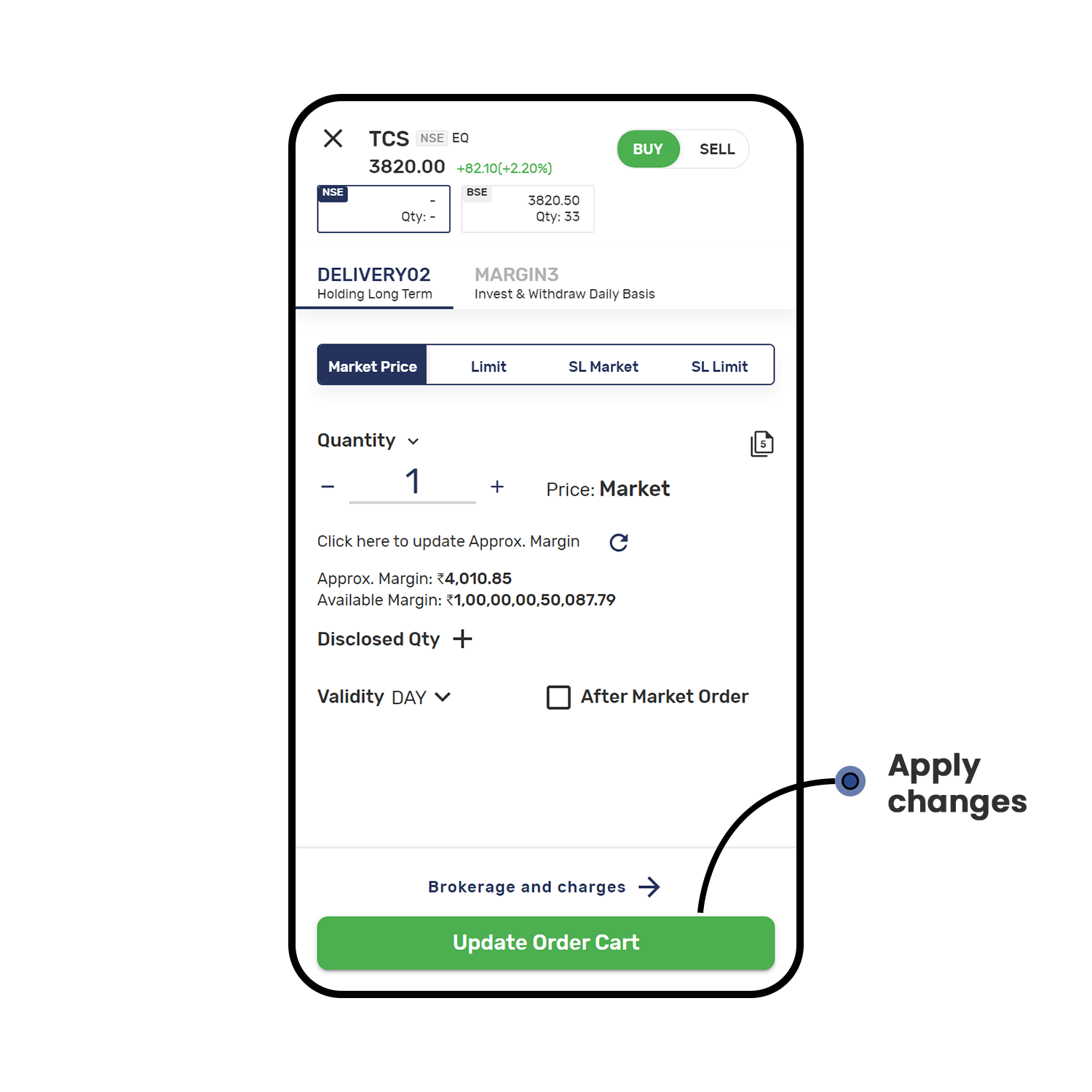The image depicts a mobile trading app interface with a rectangular shape and a black outline around it. At the top left corner, there is an 'X' icon, followed by the text "TCS." To the right, a gray area is labeled "NSEEO." Below this heading, the screen displays "3,820," with an upward trend showing an increase of 82.10 points (or +2.2%) in green text. Adjacent to this information, there are two buttons: a green "BUY" button and a white "SELL" button.

Further down the screen, two input boxes are visible. The first box appears to be for quantity, and the second is labeled "BSE," showing a value of "3,820" and a quantity of "33." Below these boxes, a section titled "Delivery 02 Holding Long Term" is underlined, indicating its heading status.

Beneath this heading, there is a segmented bar with options titled "Market," "Limit," "SL-Market," and "SL-Limit," with "Market" being highlighted in black. Following this, a quantity drop-down menu displays the number "1" set by the user. Additional details in the section include "Price Market" and an "Approximate Margin" of "4,010.65," along with an "Available Margin" field containing a numerical value. A plus sign appears next to the "Disclosed Quantity" field, and next to "Validity," there is a drop-down menu set to "Day."

At the bottom of the interface, there is a green button labeled "Update Order Cart." A line extends from this button to the text "Apply Changes," indicating further actions related to the order cart updates.